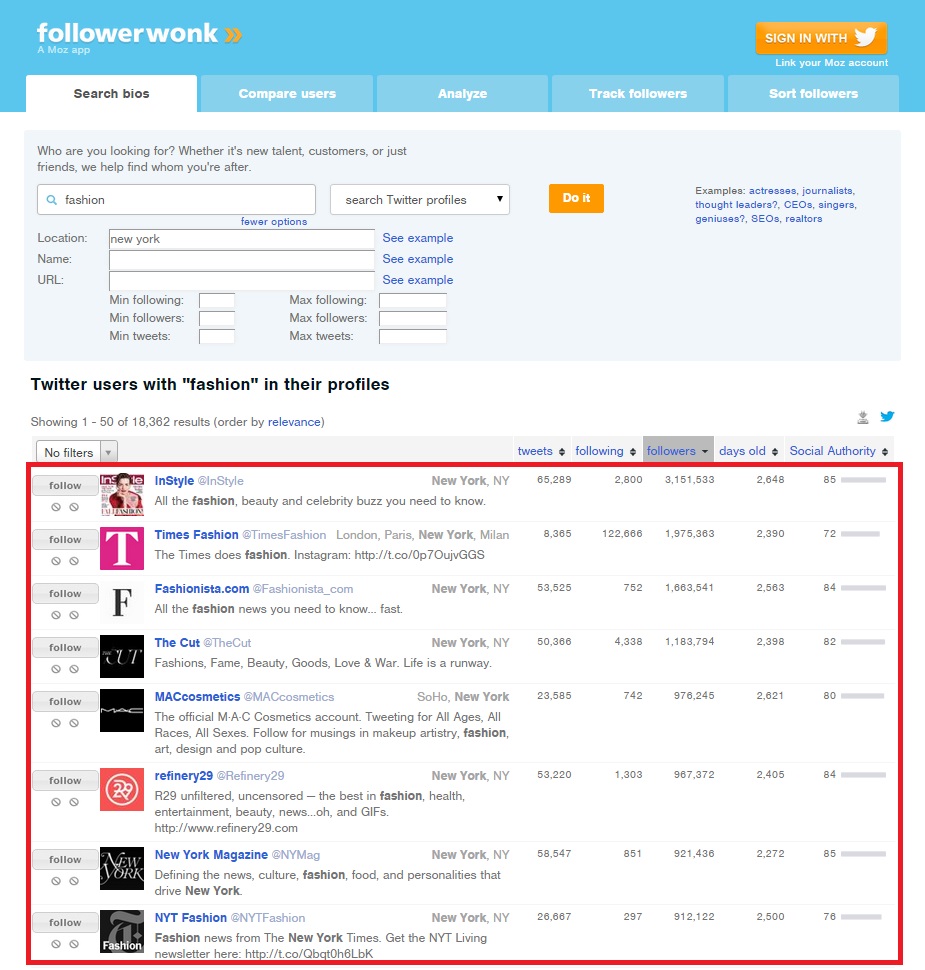The image is a screenshot taken from a desktop or laptop computer, featuring the website Followerwonk. The website's name, "Followerwonk," is prominently displayed in white text on a light blue header at the top left corner of the screen. Just below this header, the site offers five clickable tabs: "Search Bios," "Compare Users," "Analyze," "Track Followers," and "Sort Followers." The "Search Bios" tab is highlighted in white, indicating it as the current selection, while the other tabs remain in blue.

Beneath these tabs is a search box accompanied by several additional input fields where users can enter information such as location, name, and URL. Below these fields is a section displaying a list of official Twitter accounts related to fashion. This section is introduced by the caption, "Twitter users with 'fashion' in their profiles," and showcases these accounts one by one, each accompanied by its respective thumbnail icon on the left side.

A large red box has been added post-capture to highlight the entire section listing Twitter users with the keyword "fashion" in their profiles, drawing attention to this specific area for emphasis.